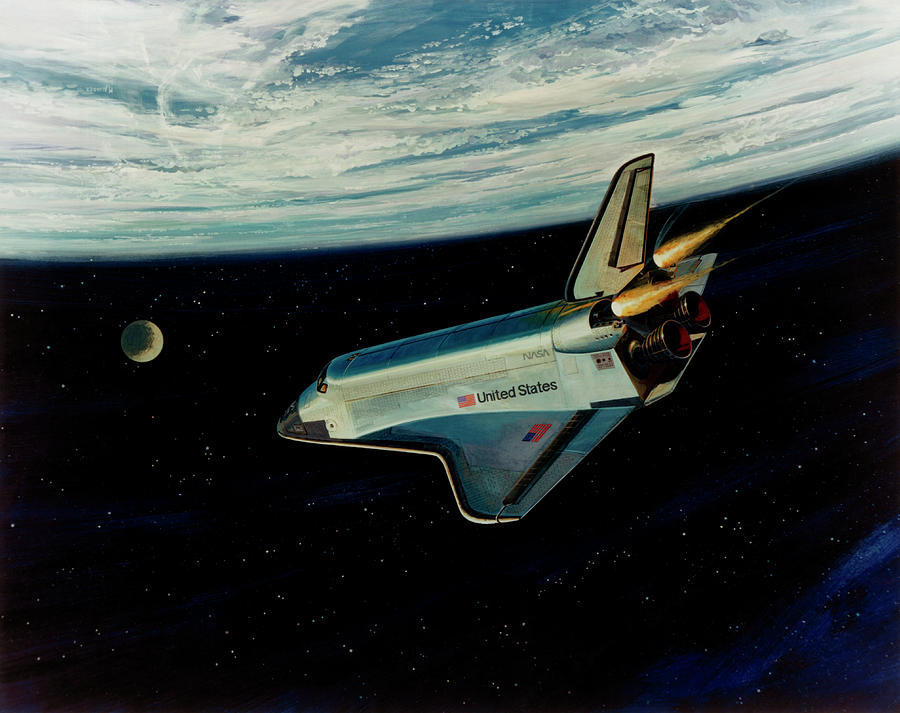The image is a detailed, hand-painted depiction of the old United States space shuttle in deep space. Dominating the top of the painting is the Earth, rendered as a "big blue marble" with visible clouds and indistinct landmasses hinting at oceans below, suggesting the view includes the South Pole. The backdrop is a vast, dark expanse of deep space, punctuated by myriad stars and a hint of the Milky Way. The moon appears to the left of the shuttle, with the rightward sun casting a shadow on its left side while illuminating the Earth above.

The spacecraft itself is painted in a silvery white hue, with "United States" and the NASA emblem prominently displayed on its side. The shuttle's gray metal body also features red, white, and blue American flag motifs on its sides and wings. The back of the shuttle showcases two larger dormant engines and two smaller ones actively emitting bright flames, indicating it's propelling through space. Its tail fin is predominantly black with gray edges.

The composition captures the shuttle appearing to swoop under the Earth, possibly nearing the space station, reminiscent of models like the Columbia. The scene evokes the technological marvel and ambition of human space exploration.